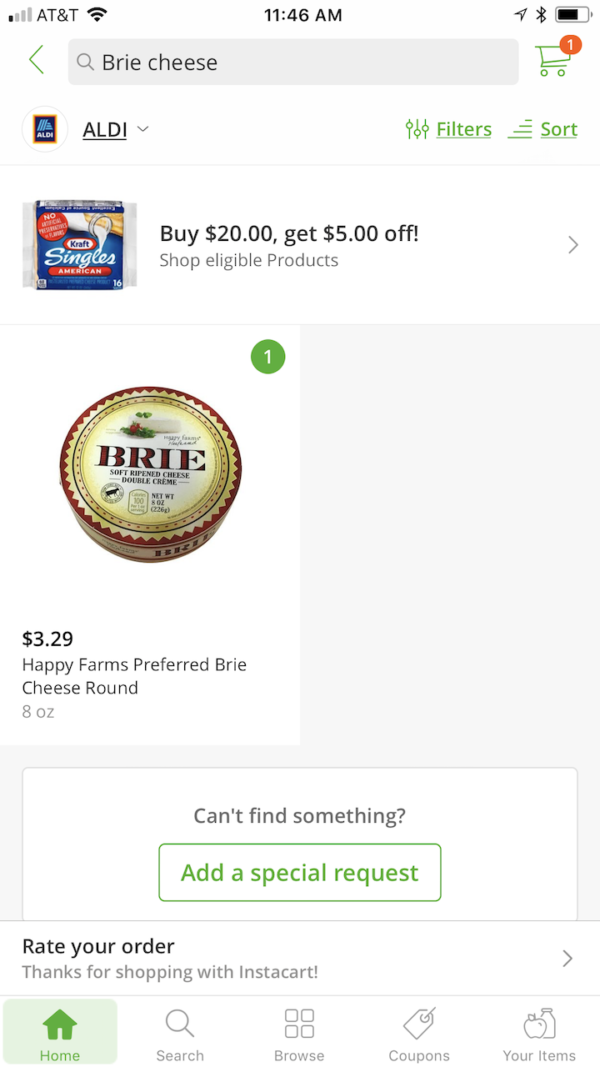The image displays a screenshot from an Instacart grocery shopping app. At the top, the status bar shows an AT&T network with one bar of signal strength, the time at 11:46 AM, and nearly full battery life. A green shopping cart icon with a red notification indicating "1" is visible alongside a search bar containing the text "Brie Cheese". A green back arrow is situated near the "Aldi" store name, accompanied by the Aldi logo in black.

Directly below, two interactive options labeled "Filter" with three horizontal lines, and "Sort" are presented. The screen features a special offer: "Buy $20, get $5 off," with a prompt to "Shop eligible products". 

The main product listed is "Happy Farms Preferred Brie Cheese Round, 8 ounces" priced at $3.29, highlighted with a red and yellow label and marked with a green quantity indicator "1".

Further down, a section prompts users with "Can't find something?" followed by a green button labeled "Add a special request". Below this, it reads "Rate your order" and "Thank you for shopping with Instacart" in black text. The navigation bar at the bottom has a green highlighted home button, while "Search," "Browse," "Coupons," and "Your Items" remain unselected in gray.